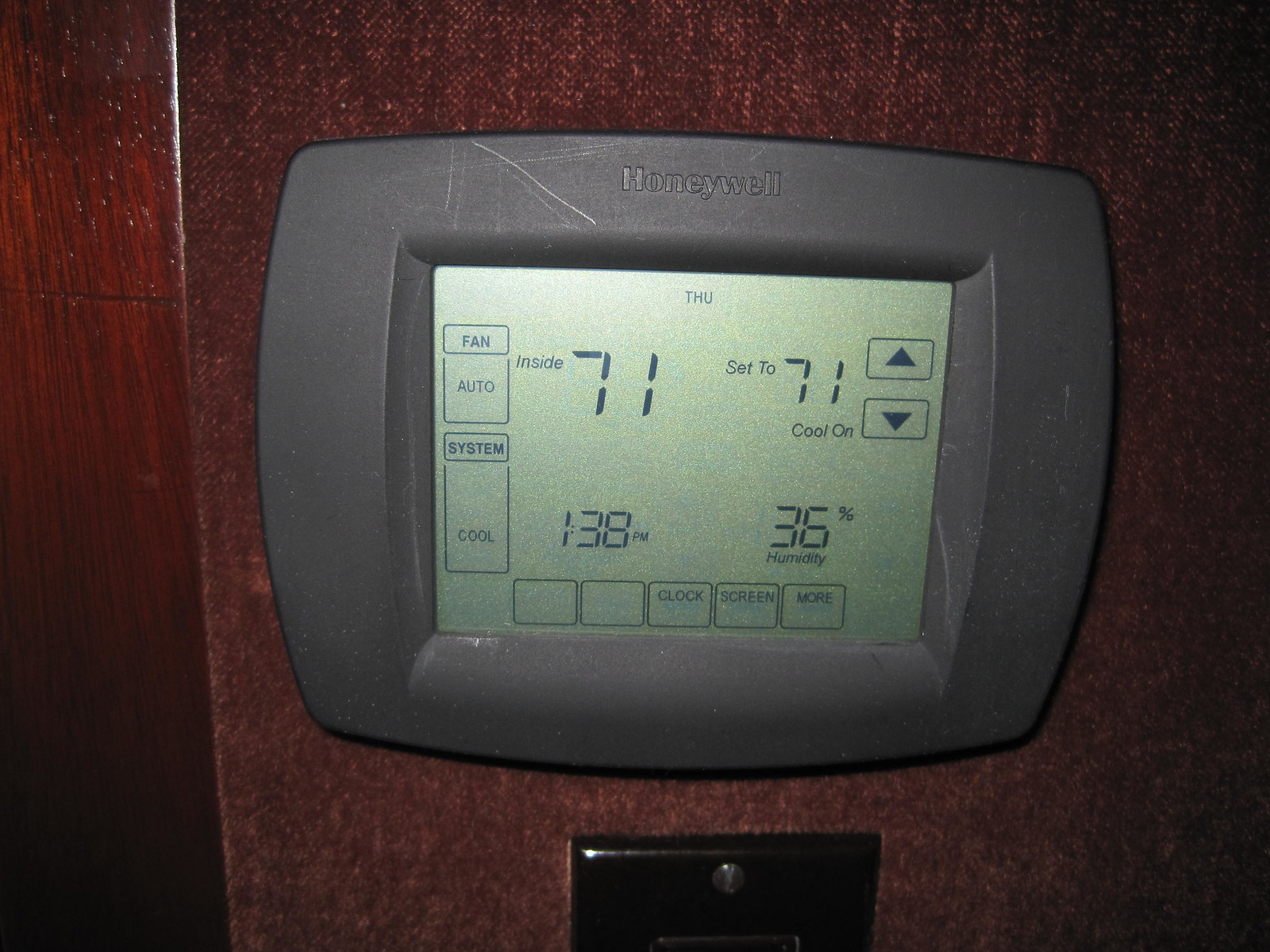This close-up photograph features a Honeywell electronic thermostat prominently mounted on a brown wall. The thermostat interface, encased within a grey plastic cover, displays various settings and readings. 

To the left of the thermostat, a dark reddish-brown wooden door frame is partially visible. Below the thermostat, the top portion of a light switch is discernible. 

The interface of the Honeywell thermostat shows 'Fan Auto' at the top left and 'System Cool' beneath it. At the top center, the display indicates the day as 'THU' (Thursday). The interior temperature reads 'Inside 71', with 'set to' appearing alongside it. The screen also shows 'Cool On' accompanied by two black arrowheads, one pointing up and one down. 

Further details include the current time, '1:38 PM', and the humidity level, '36%'. At the bottom of the interface, five blocks are shown; the first two are empty, followed by labels 'Clock', 'Screen', and 'More' respectively in the other blocks.